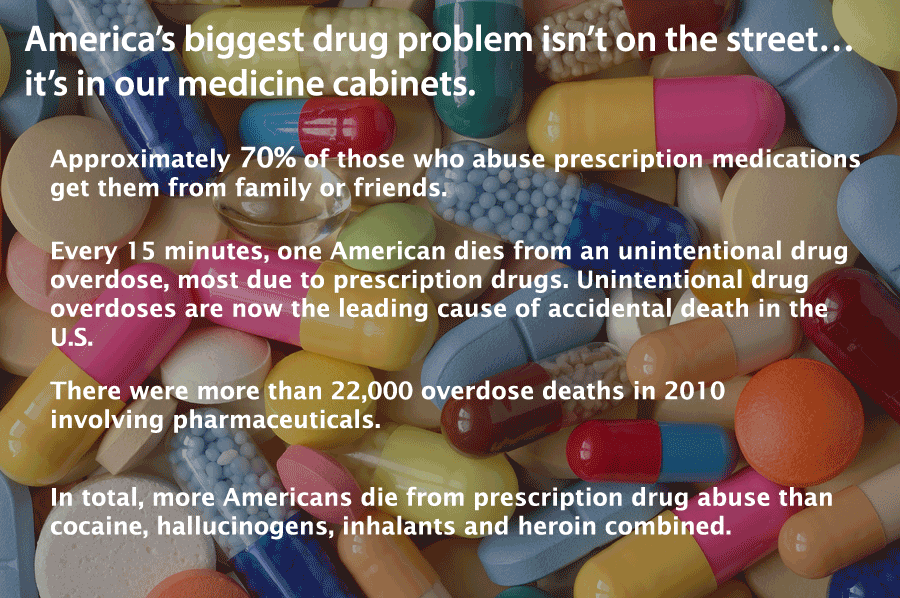The image is a rectangular PowerPoint slide with the long sides on top and bottom, featuring a close-up background of various colorful pills resembling candy. The pills include blue capsules, pink and yellow capsules, green, pink, blue, red, turquoise, and orange round pills, along with oval and caplet shapes. Prominently, in bold white text at the top, the slide reads, "America's biggest drug problem isn't on the street... it's in our medicine cabinets." The infographics continue with alarming statistics: "Approximately 70% of those who abuse prescription medication get them from family or friends. Every 15 minutes, one American dies from an unintentional drug overdose, most due to prescription drugs. Unintentional drug overdoses are now the leading cause of accidental death in the U.S. There were more than 22,000 overdose deaths in 2010 involving pharmaceuticals. In total, more Americans die from prescription drug abuse than cocaine, hallucinogens, inhalants, and heroin combined." The carefully designed slide highlights the pervasive issue of prescription drug abuse in the United States, emphasizing its hidden presence in everyday household medicine cabinets.